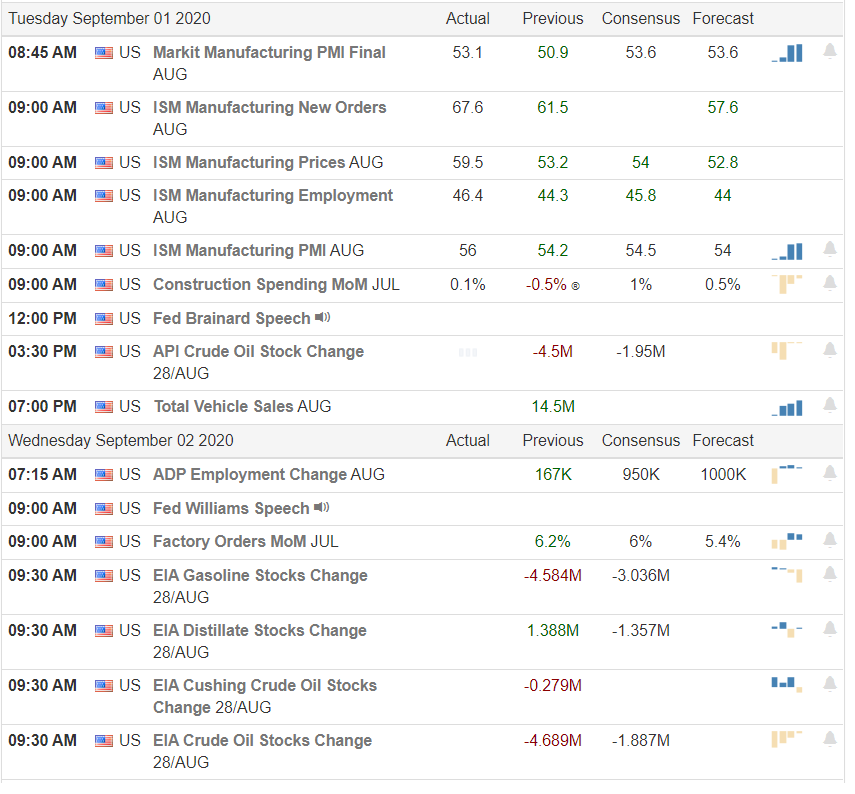This is a detailed analysis of a financial data website displaying various economic indicators and figures for a specific date, Tuesday, September 1st, 2020. The table is organized into columns—Actual, Previous, Consensus, and Forecast—providing a comprehensive overview of economic activities. Notable entries include:

- **8:45 AM:** U.S. Market Manufacturing PMI (Final for August)
  - Actual: 53.1
  - Previous: 50.9
  - Consensus: 53.6
  - Forecast: 53.6

- **9:00 AM Onwards:** Various economic indicators such as new orders and prices are listed, continuing up to 7:00 PM.

At 7:00 PM, the table specifies:
- **Total Vehicle Sales for August:** 14.5 units

For Wednesday, September 2nd, 2020, the table similarly lists economic indicators with different events such as:
- **ADP Employment Change**
- **Speech by Bette Williams**

This website appears to cater to tracking and forecasting economic performances on a daily basis, providing critical financial insights for each indicator.